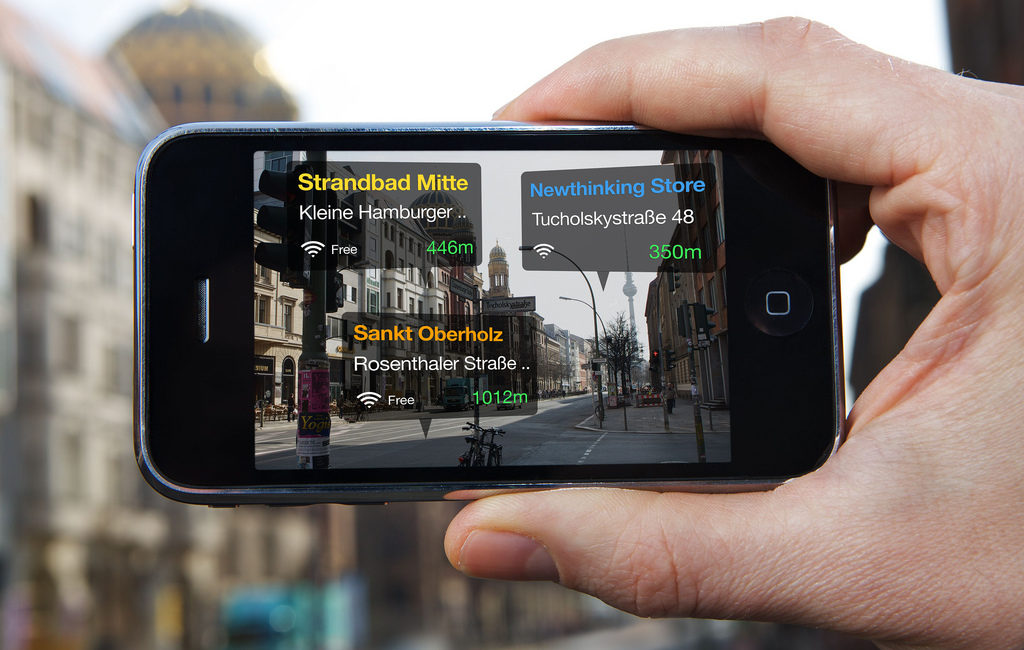In this colorful and brightly lit image, a detailed scene unfolds with a hand extending from the right side, holding an iPhone in landscape mode. The hand, prominently featured with visible wrinkles and striations, grips the relatively small, black phone with silver trim. The thumb is positioned at the bottom, while the fingers rest on top. The iPhone screen is illuminated, displaying a street scene with tall buildings on either side, captured from a road view. The phone's interface overlays text onto the image, identifying surrounding structures and their distances: "Strand Bad MITI Klein Hamburger" at 446 meters on the top left, "New Thinking Store to Close Skystripe 48" at 350 meters on the top right, and "Sanct Overhauls Rosenholmer Strab" at 1012 meters at the bottom. The hand-held device seems to be using an augmented reality application to annotate the real-world environment, as evidenced by the matching but out-of-focus background visible behind the phone.